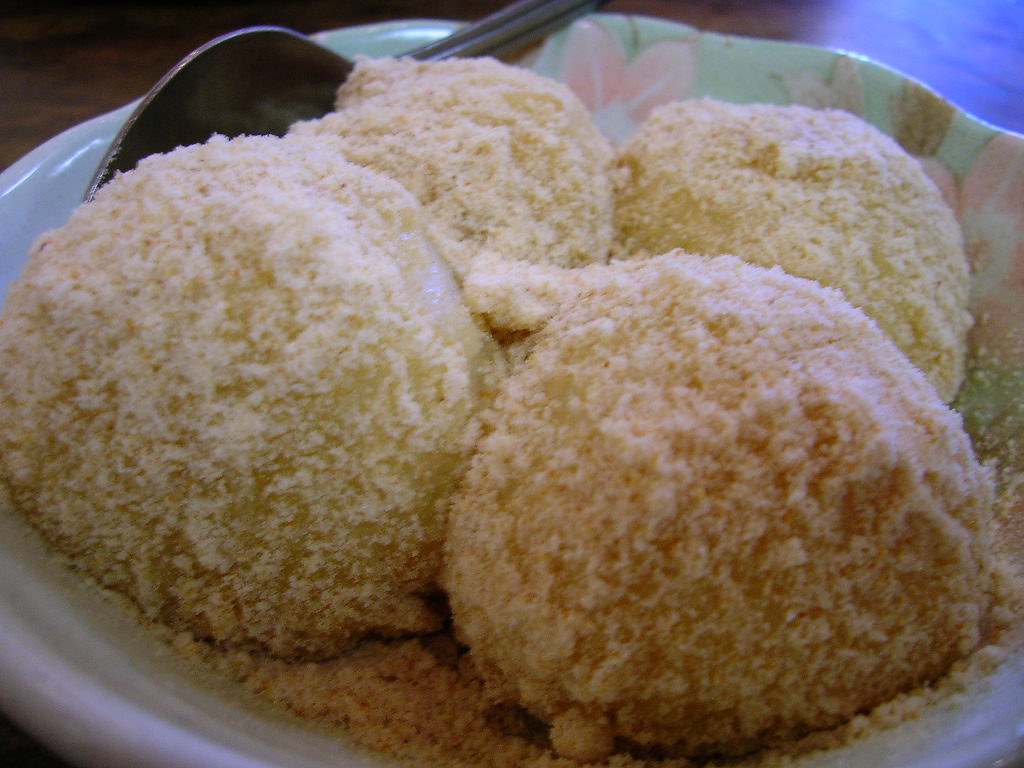The image depicts a close-up of a wavy, rectangular bowl resting on a dark wooden surface that reflects light in the top right corner. The bowl itself is light green with delicate pale pink flowers and green leaves decorating its interior. In the top left corner, a large silver spoon with a slightly purple hue is resting inside the bowl, its handle extending out to the right. The bowl contains four round, doughy, off-white spheres covered in a fine powder that looks like breadcrumbs or perhaps a sweet sugar concoction. The bottom of the bowl is sprinkled with a layer of what appears to be light brown sugar, adding to the overall texture of the dish.